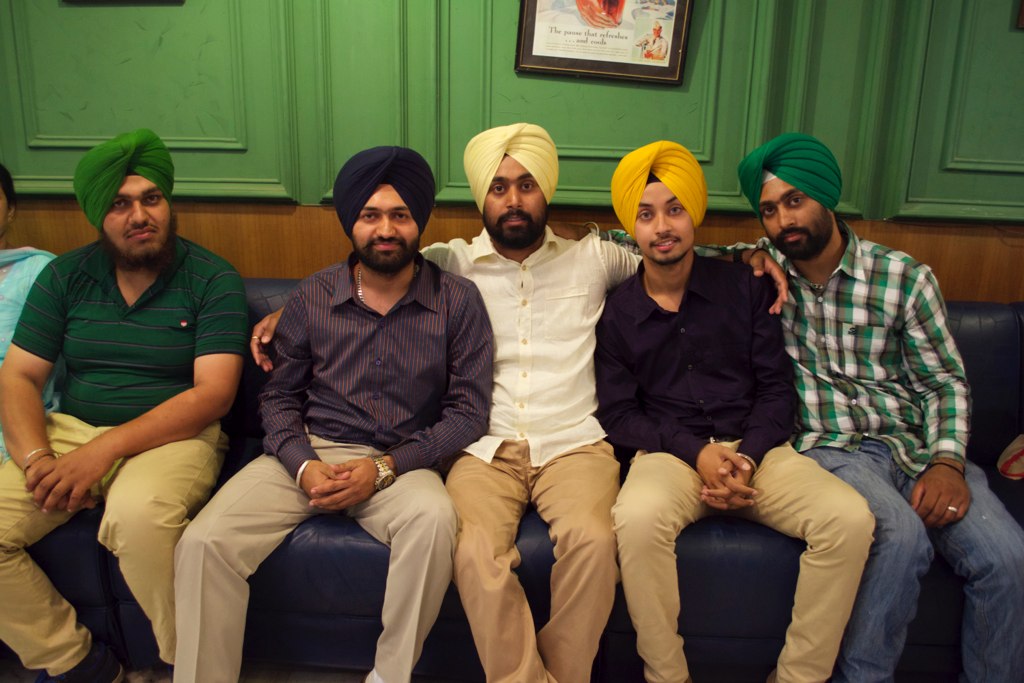The photograph features five men of Middle Eastern descent, seated closely together on a blue leather sofa, against a green and brown wall backdrop. From left to right:

- The first man has a tanned complexion, a black beard, and a green turban. He sports a green polo shirt paired with khaki pants and rests his hands in his lap. He wears a watch on his right wrist.
  
- The second man, also with a dark tanned complexion and facial hair, dons a purple button-down shirt and light brown dress pants. His turban is navy blue. He has a watch on his left wrist.

- The central man anchors the group with his arms wrapped around the shoulders of the men next to him. He is dressed in a white button-down shirt with khaki pants and a cream-colored turban.

- The fourth man, maintaining the relaxed ensemble, wears a yellow turban, a long-sleeved black (or dark-colored) button-down shirt, and khaki pants. He has minimal facial hair, notably a small mustache and beard growth under his chin.

- The man on the far right completes the row wearing a green plaid flannel shirt with shades of white and gray, denim jeans, and a green-colored turban. He, too, has darker tanned skin and facial hair.

Above the men, a slightly tilted brown picture frame hangs on the green part of the wall, with unclear contents incorporating white, pink, and blue hues. All the men sit comfortably, looking directly at the camera, exuding a casual and connected vibe.